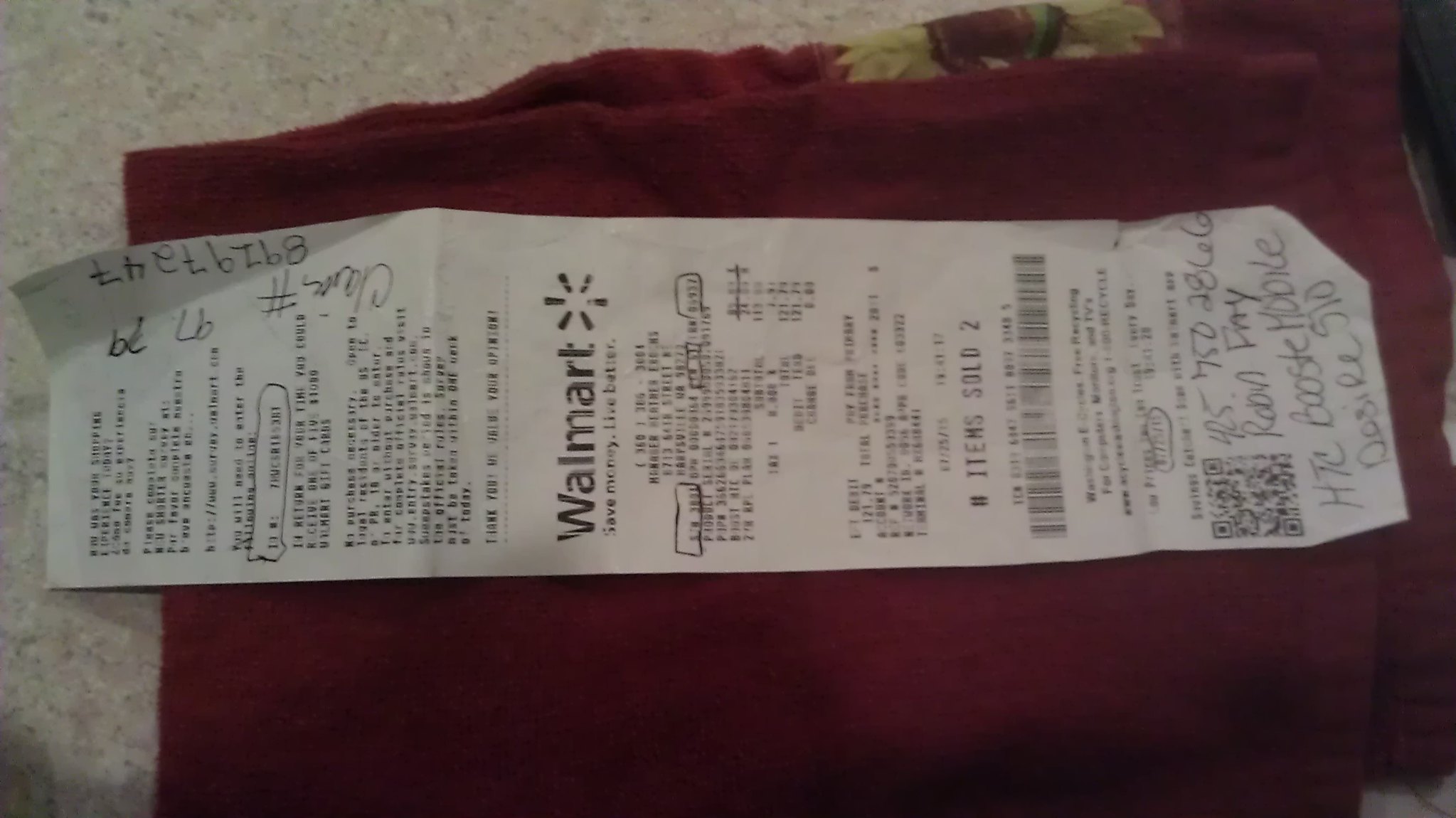In this horizontally oriented rectangular image, a tan granite countertop serves as the backdrop. Resting on the countertop is a neatly folded burgundy towel. Positioned atop the burgundy towel is a horizontally laid white receipt. The receipt prominently features the Wal-Mart logo, complete with their iconic six-pointed star, printed in black ink. Beside the logo, some text is discernible, though much of it appears too small or faded to fully interpret. Notably, the words "items sold: two" stand out. Additionally, there is a barcode located on the lower left side of the receipt. Handwritten in black ink near the scan code are the words "Robin Fay HTC Boost Mobile."